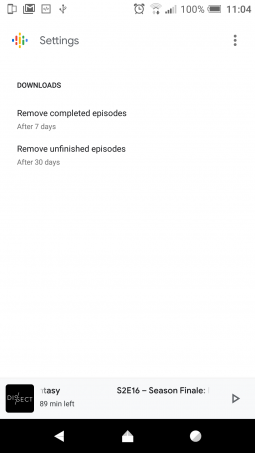This image is a screenshot of a settings page, displaying a clean and organized interface. At the top left corner, the word "Settings" is prominently displayed, accompanied by a distinctive diamond-shaped logo adjacent to it. This logo is composed of bars in various colors: blue, red, yellow, green, and another blue bar.

Underneath the heading, there is a section labeled "Downloads." This section contains two specific settings: "Remove completed episodes after 7 days" and "Remove unfinished episodes after 30 days," providing clear options for managing downloaded content.

At the bottom of the screen, a video player interface is visible, set against a gray bar. The current episode displayed is titled "S2E16 Season Finale." The interface includes a play button positioned on the right side and a thumbnail image on the left.

At the very top of the screenshot, the phone's user interface is also visible, indicating a 100% battery level and the time as 11:04, all set against a white background.